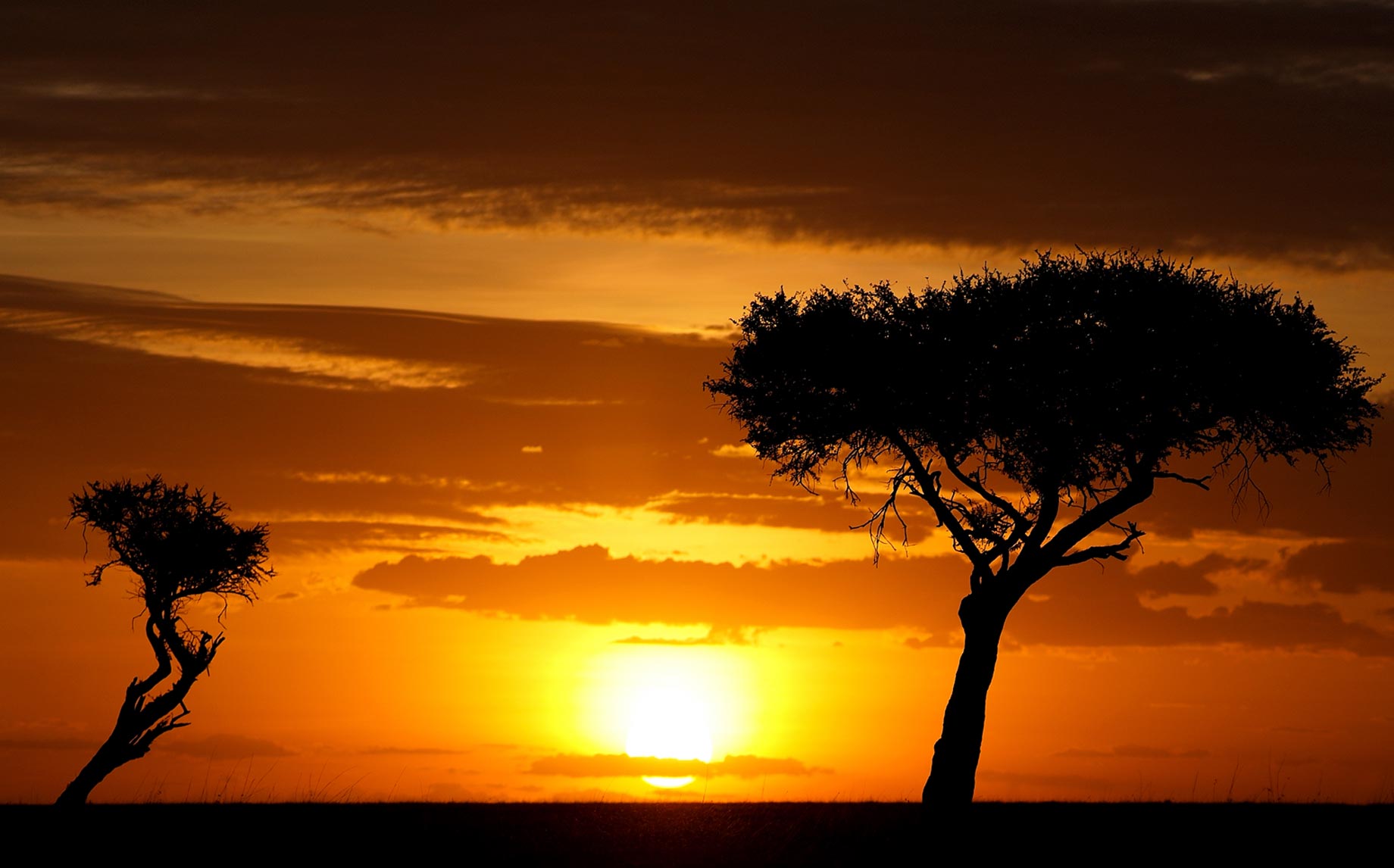A color photograph in landscape orientation captures a dramatic sunset over a flat, arid landscape, reminiscent of the African Serengeti. The sky's vivid hues transition from burnt orange at the top to a bright, fiery yellow around the nearly-set sun, which is a bright white circle at the horizon. Wispy, horizontal bands of purple clouds adorn the upper and middle sections of the sky, enhancing the striking sunset colors. The foreground features two silhouetted trees: the left tree is smaller, with sparse gnarly branches and a small, bushy canopy, slightly tilting to the right. In contrast, the right tree is taller, with a fuller, flattish canopy and a sturdier trunk, also leaning gently to the right. A thin, black strip across the bottom of the image represents the flat ground, completing this vivid representation of a serene, quintessential African sunset.